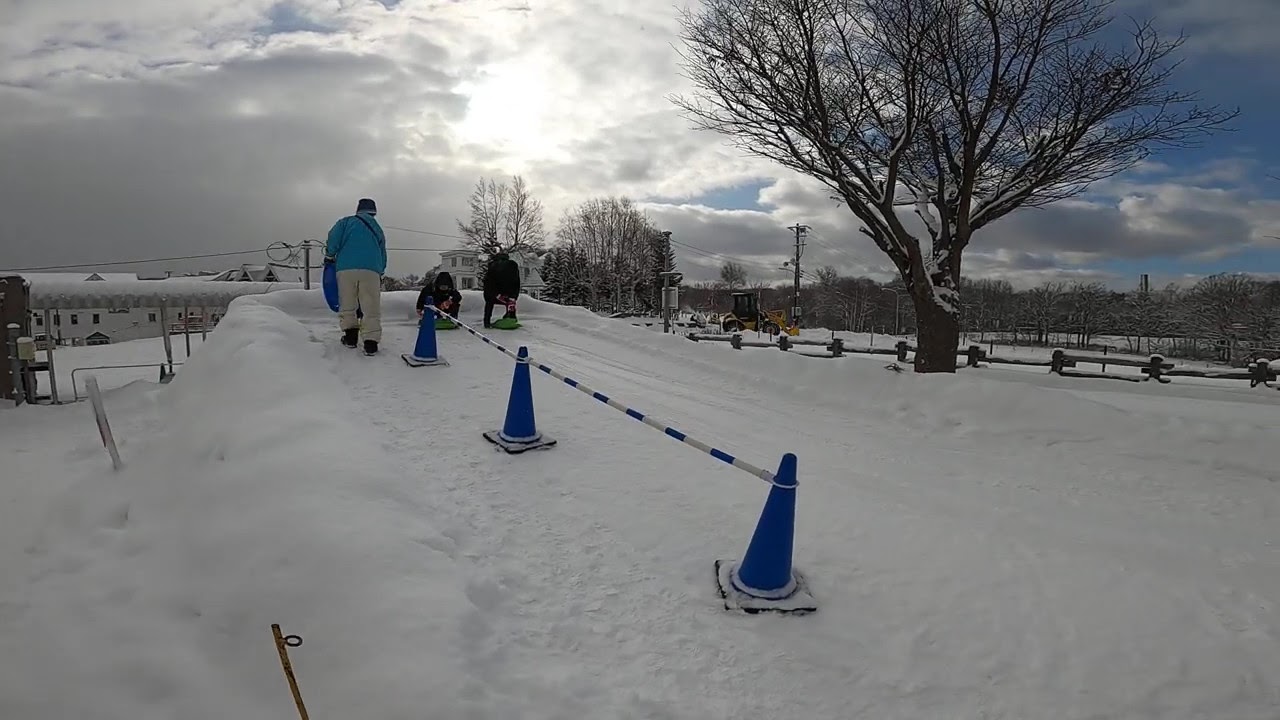This photograph captures a snowy scene set in what seems to be a suburban park. Dominating the image is a snowy slope that serves as a makeshift sledding track, marked by three blue traffic cones interconnected with racing stripes. At the base of the slope, the ground is blanketed in a thick layer of pure white snow. In the middle ground, three young children, dressed warmly in winter attire including black and turquoise jackets, are preparing to sled down the hill. Two of the children, with sleds resembling boogie boards, stand ready to slide, while another child, in a blue jacket and cream-colored pants, trudges up the hill, possibly officiating or supervising the race.

To the left and center of the image, a barren tree with snow-dusted branches stands prominently. Behind this tree, the backdrop features a wooden fence also covered in snow, and further back, distant apartment buildings peek out. To the right, more leafless trees stretch into the cloudy, mostly gray sky. Though the sun attempts to break through the cloud cover, it remains mostly concealed, casting a subdued light over the entire scene. The photo captures a moment of joyous anticipation as the children gear up for the thrill of descending down the snowy slope.